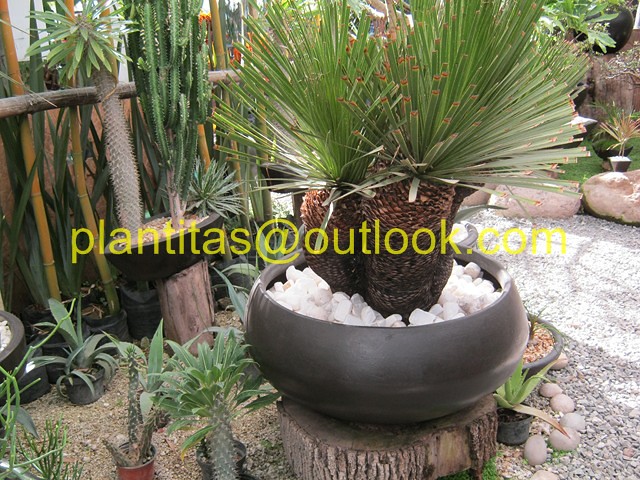In this horizontally long, daytime photograph of a southwestern-style garden, a variety of desert plants are artistically arranged. At the forefront stands a striking palm-like plant, housed in a short, wide, gray clay bowl filled with white rocks. This distinctive plant features a thick, scaly trunk reminiscent of fish scales, topped with grass-like green fronds. Surrounding this main plant are an assortment of cacti and succulents, each adding unique textures and shapes to the scene. Notably, a spiky, woody-looking cactus stands prominently among other plants with cucumber-shaped forms and grass-like appearances. To the left, a black pot holds a plant with a pineapple-like configuration. The garden also features a pathway crafted from white stones that curves to the right, bordered by a few substantial rocks. In the upper right corner, a cluster of large white stones enhances the rustic, natural ambiance of the setting.